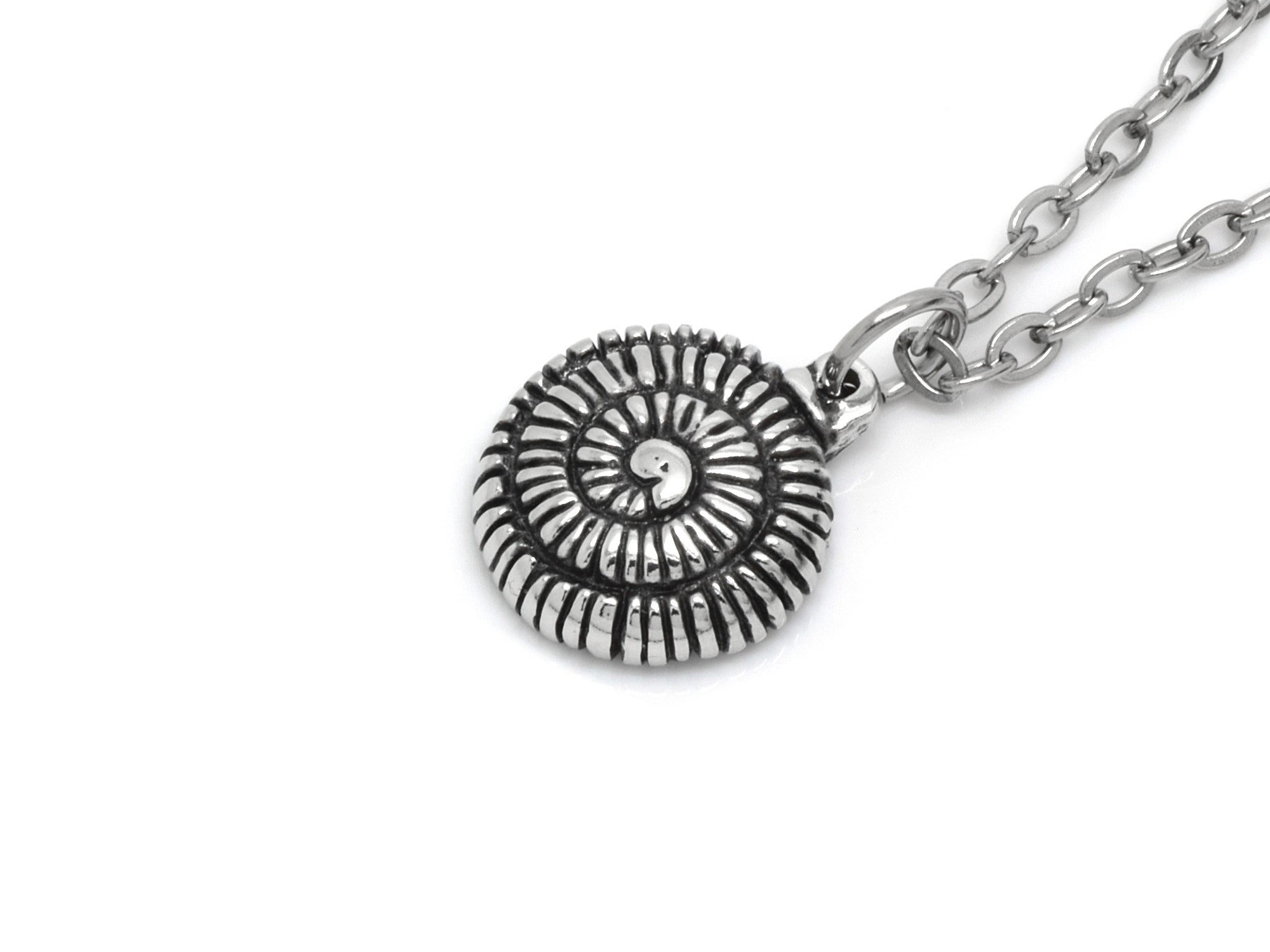This is a detailed photograph of a necklace, meticulously centered against a simple, solid white background. The photo captures a striking medallion shaped like a tightly coiled snake, with its head nestled in the center and its tail looping underneath to connect with a silver hook. The snake medallion is predominantly silver, accentuated by black cracks and deep borders that give it a rich, textured appearance. This intricate spiral structure is composed of numerous silver lines, each separated by defined black lines, creating a segmented, almost sliced visual effect. Only part of the silver link chain is visible, emerging from the top right corner to attach to the loop holding the medallion. Overall, the image showcases the detailed craftsmanship of the necklace's silver and black accents against the contrasting white backdrop.